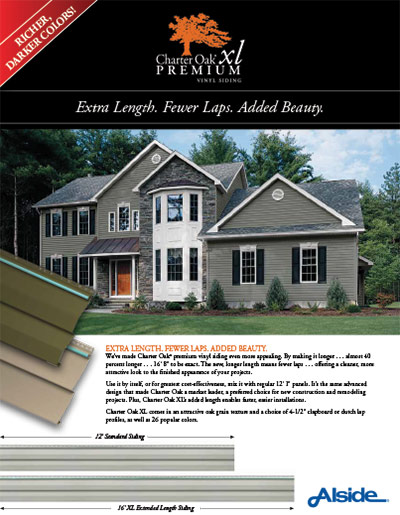### Detailed Caption:

This image is an advertisement for a company specializing in premium vinyl siding. The upper left corner of the ad features the text "Richer, Darker Colors" set against a striking red background. At the top of the page, a black banner stretches across, showcasing an image of a vibrant orange oak tree. Directly below this image, white text reads: "Charter Oak XL Premium Vinyl Siding." Further down, additional text highlights the benefits: "Extra Length, Fewer Laps, Added Beauty."

Dominating the central portion of the ad is a detailed photograph of a gray, two-story house front. The home features several windows and a welcoming porch leading up to the front door. Adjacent to the house image, two samples of siding are displayed — one in green and the other in tan hues.

The descriptive text states: "We've made Charter Oak Premium Vinyl Siding even more appealing by making it longer — almost 40% longer, 16 feet 8 inches to be exact. The new longer length means fewer laps, offering a cleaner, more attractive look to the finished appearance of your projects."

Additional technical product details follow. An illustrated comparison underneath features three sections of siding: a 12-inch standard piece, a 12-foot standard piece, and a 16-foot selection of extra-large, extended-length siding. To the right, in striking blue text, is the company name: "Alside."